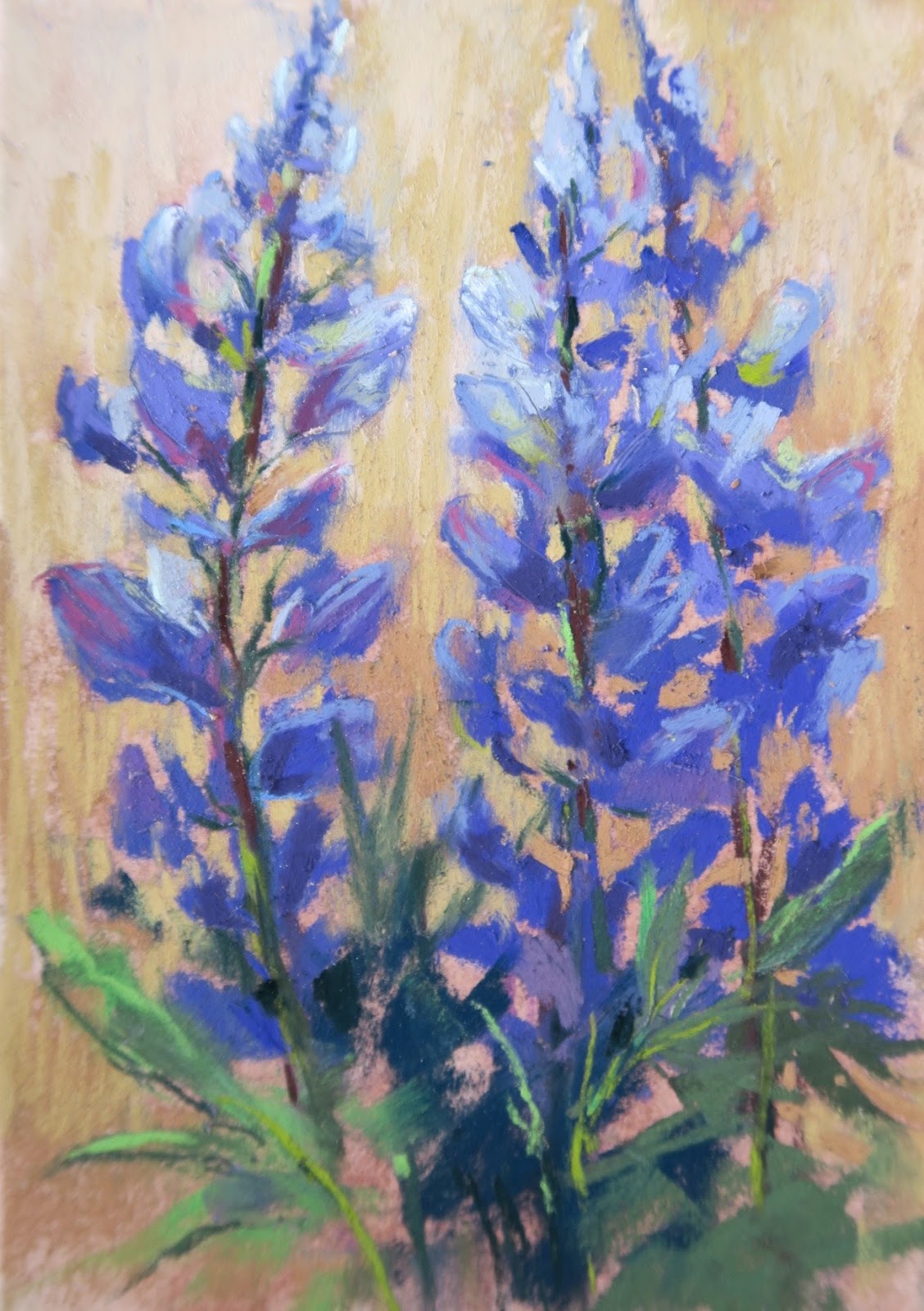The image is a painting, possibly watercolor, depicting three tall-stemmed flowers that may be forget-me-nots, foxgloves, or delphiniums. These flowers are arranged in a bouquet, with each stem adorned with numerous small, tapering blue petals that vary in shade from light to dark blue, and some even have touches of yellow and purple. The stems at the bottom are dark brown, transitioning upwards into a cluster of leaves in varying shades of green, from lime to darker hues. The background is a soft, pinkish beige that allows the flowers to stand out starkly, reinforcing them as the central focus of the painting. The delicate use of color and shading, including hints of reds and uses of blacks in the stems and base, enhances the overall texture and depth of the floral composition.